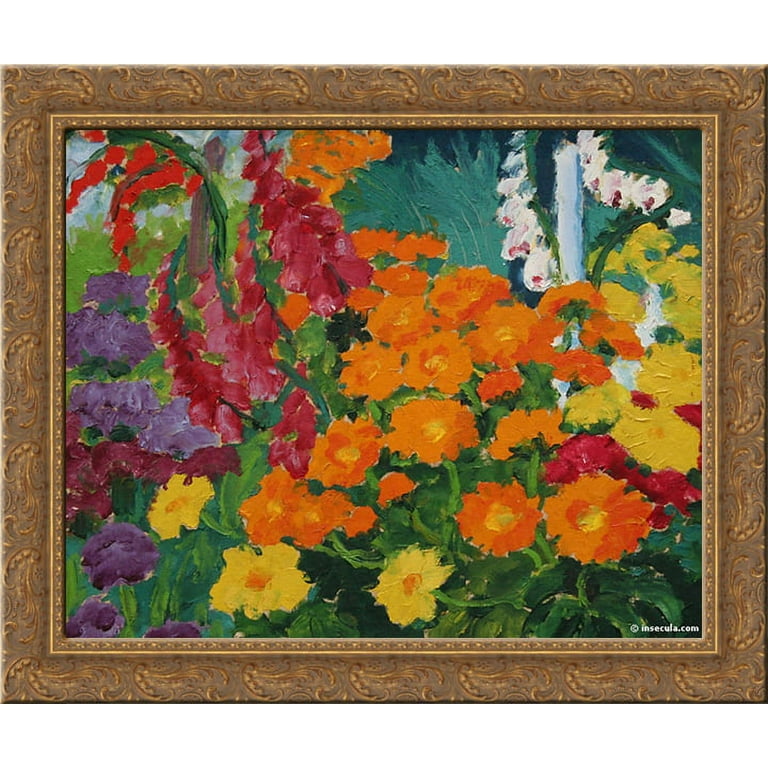This image features a digitally rendered mock-up of a painting displayed against a stark white background. The painting is set within an ornate, Baroque-inspired frame that has a brass or gold appearance with elaborate filigree designs. The focus of the painting is a vibrant array of flowers depicted in an impressionist style, where the subjects are identifiable but not photorealistic.

At the center of the painting, a large bouquet of marigold-shaped orange flowers is surrounded by similarly shaped yellow flowers. Among them, along the left edge, tall spikes resembling foxgloves in a burgundy hue stand out. Dark purple flowers, possibly resembling poppies, are visible along the sides, with some red vine-like flowers intertwined.

The backdrop of the painting is punctuated by various shades of green representing shrubs, trees, or grass. A hint of blue sky is visible in the top left corner, adding a touch of landscape to the floral composition. The bottom right corner of the painting bears a small white text that reads "insecula.com," indicating a digital watermark or copyright signature.